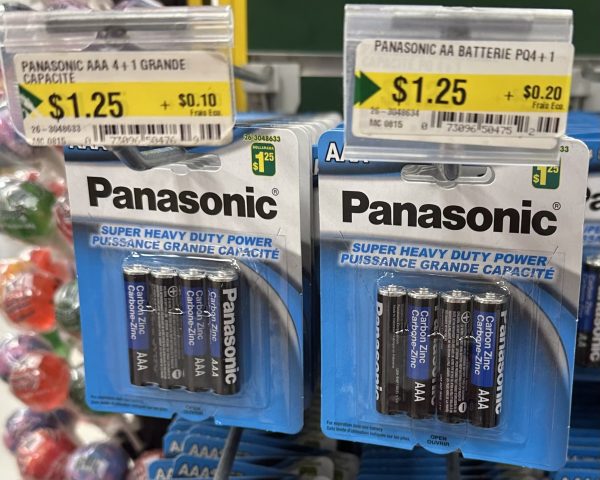This vibrant color photograph, taken inside a store, meticulously showcases a prominently displayed rack of Panasonic batteries. Dominating the central portion of the image are two packages of Panasonic AAA Super Heavy Duty Power batteries, each containing four batteries. The packages are neatly suspended from a wire rod, with a plethora of identical packages hung behind them. Each package front reads “Panasonic Super Heavy Duty Power Puissance Grande Capacité,” with a small plastic tag affixed above, detailing "Panasonic AAA 4 Plus 1 Grande Capacité, $1.25 plus $0.10." Adjacently, in the bottom left corner, a blurry yet distinguishable assortment of red and green lollipops are for sale, adding a splash of color contrast. The lower portion of the photograph hints at an extended rack of batteries that stretches out of the frame. Notably, the image is devoid of people, animals, or any vegetation, focusing solely on the neatly arranged display of products within the store's interior.